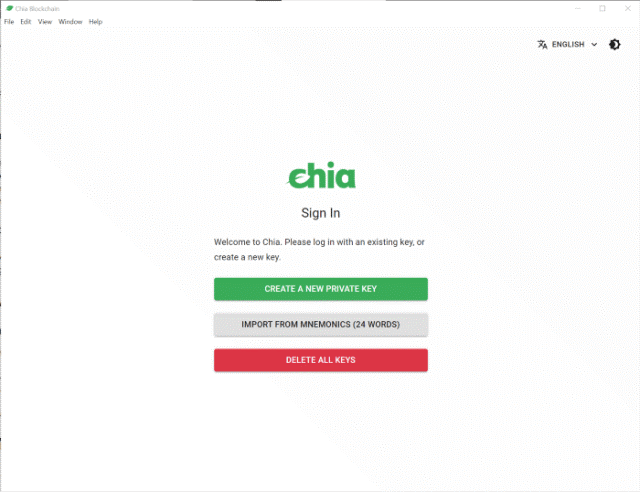The image is a detailed screenshot of a white, rectangular webpage for the Chia sign-in page, primarily in English. In the top left corner of the page, there are the options: File, Edit, View, Window, and Help in black text. The upper right corner displays the word "English" with a down arrow next to it, indicating a drop-down menu, along with an icon to toggle between light and dark modes.

Center-aligned, the Chia logo is prominently displayed in green, with a distinctive white leaf through the letter "C." Below this, the word "Sign In" appears in black, followed by the greeting "Welcome to Chia. Please log in with an existing key or create a new key." Users have three action buttons beneath this message. The first button says "Create a New Private Key" in white text on a green background. The second button, "Import from Mnemonics (24 words)," is in black text on a gray background. The third option, "Delete All Keys," appears in white text on a red background. The overall background of the page is white, and the design elements are centrally located. The screenshot depicts the initial interface for registering or signing into a Chia account, emphasizing the options for key management.